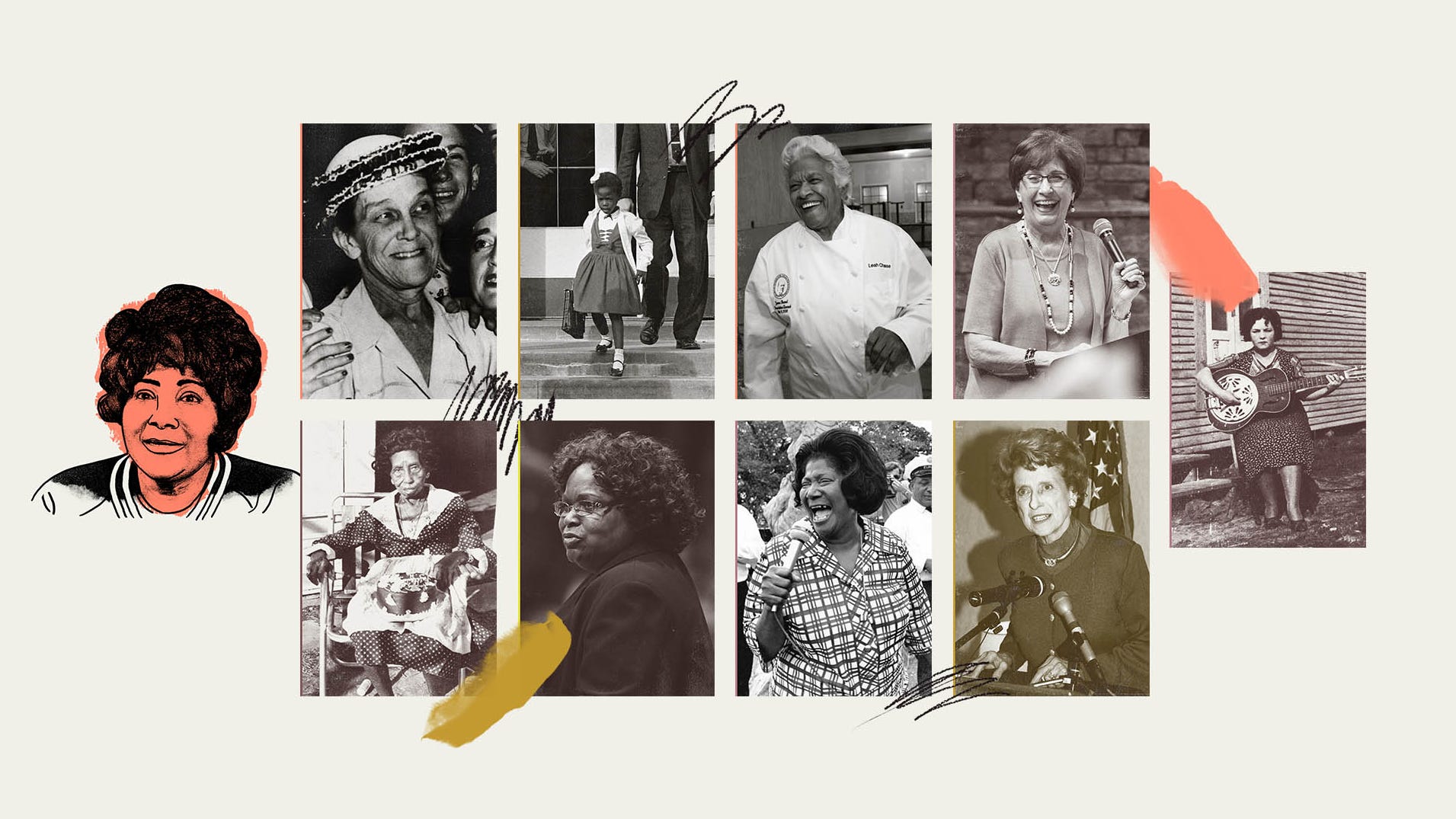This image, set against an off-white background, is a montage of ten distinct pictures showcasing significant women in history, primarily focusing on African-American figures, alongside a few White women. On the far left, a detailed black and white sketch depicts an African-American woman with short hair, framed by an orange background. To the right, a grid of eight photographs is arranged in two rows of four. The top row begins with an elderly gentleman surrounded by smiling people, followed by a young African-American girl, likely one of the first children to integrate into schools, walking down stairs with a suited man behind her, possibly an officer. Next, a smiling chef in a white uniform is featured, and the row ends with a woman laughing and holding a microphone, adorned in short hair, glasses, and a dress suit. The bottom row starts with an elderly African-American woman in a floral dress sitting on a chair, followed by another woman with short curly hair and glasses. The third image captures a woman, resembling Aretha Franklin, laughing into a microphone, dressed in a floral outfit. The row concludes with a woman who appears to be Nancy Reagan, standing in front of microphones with the American flag in the backdrop. On the far right, a young woman, possibly in her early twenties, is seated on a stump playing a banjo or guitar in front of a wooden house. The collection distinctly highlights the diverse, impactful roles these women and others have played in history.